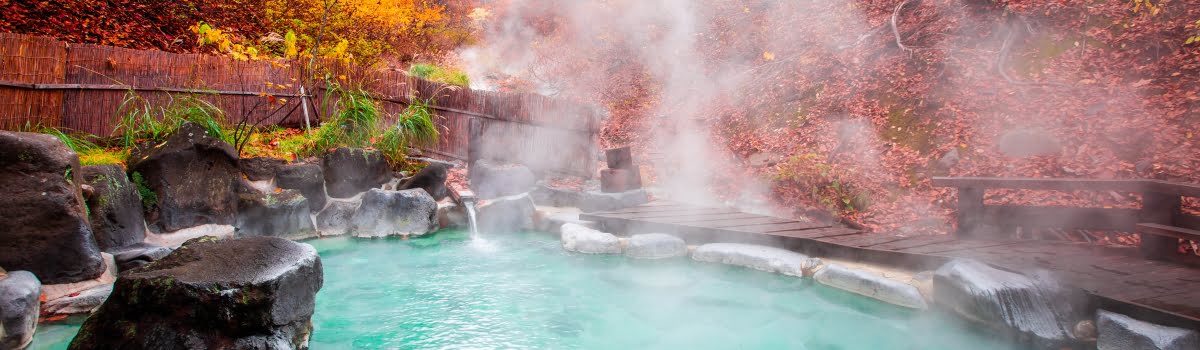The image depicts a tranquil outdoor setting, resembling a natural hot spring or a heated man-made pool designed to emulate one. The scene is captured in a wide, panoramic photograph featuring a long, rectangular pool of light, translucent teal water, from which steam gently rises, indicating its warmth. The pool is bordered by white and gray stones, creating a natural, inviting edge. To the right, a dark brown wooden walkway extends, accompanied by a partial railing that eventually gives way to an open section. Beyond this walkway, a hillside is visible, adorned with a mix of green grass and fallen red leaves, indicative of autumn. Bushes dot the landscape, enhancing the natural feel. On the left side, a rustic wooden fence, displaying hues of yellow, red, and brown foliage, runs parallel to the pool, delineating the space. Additional trees with shades of pink, orange, and yellow foliage, and some green shrubbery further enrich the serene, cozy ambiance of the scene.